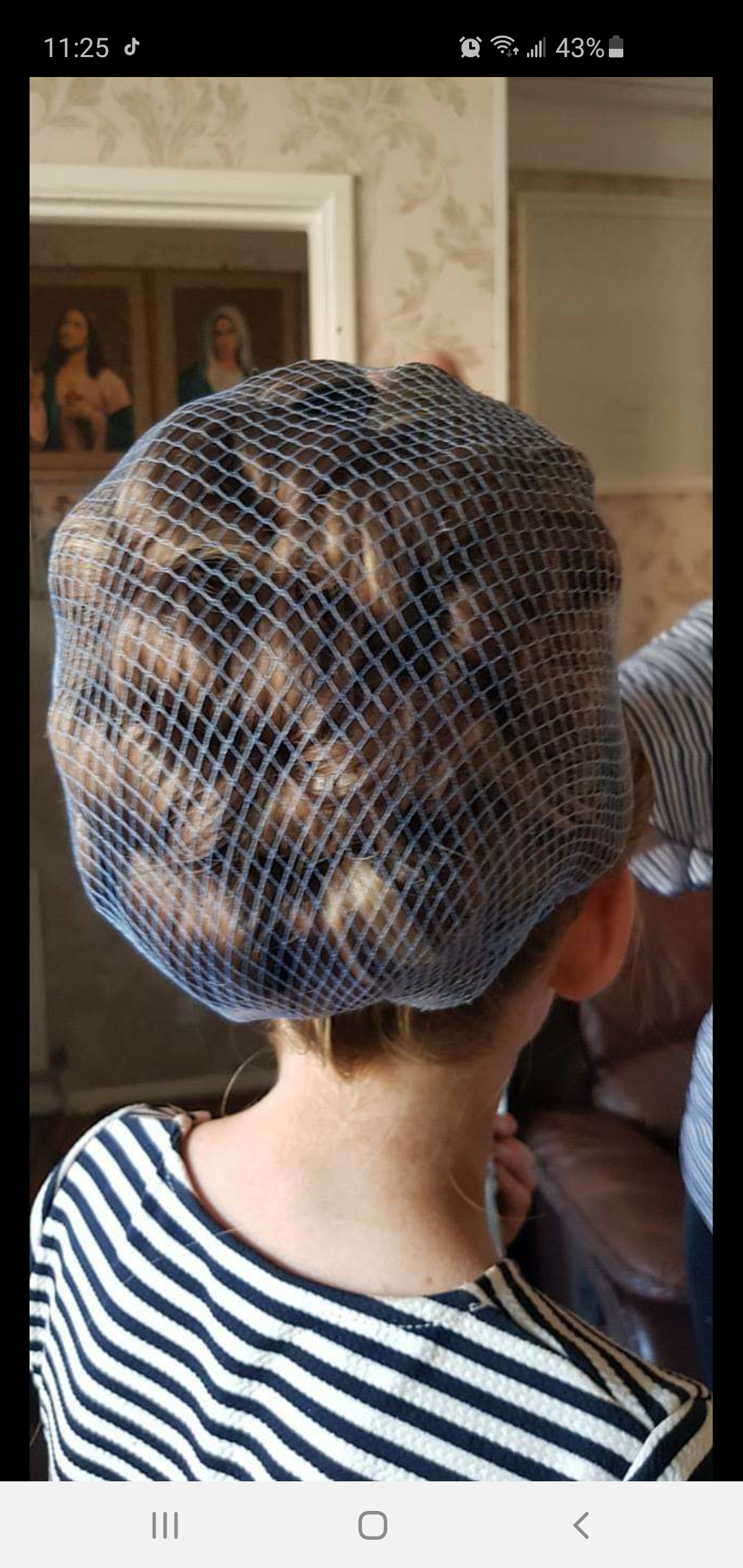The image is a screenshot depicted on a phone, with a black banner framing the sides and top. At the top right corner, the time reads 11:25 in white text. Various symbols are visible: a white TikTok icon, an alarm symbol, a Wi-Fi signal indicator, a cellular signal icon, the battery percentage at 43%, and a battery icon. The bottom banner is white, featuring three gray lines, a gray square, and a left-pointing arrow.

The main image shows the back of a child’s head, with light skin and golden, curly hair secured with a blue hairnet. The child is wearing a blue and white striped shirt. In the background, there is a room with tan wallpaper adorned with Victorian-looking portraits and images of Jesus and Mary. The wallpaper has vine etchings, and part of a person’s arm is visible, suggesting they might be attending to the child’s hair, possibly in a beauty shop setting.